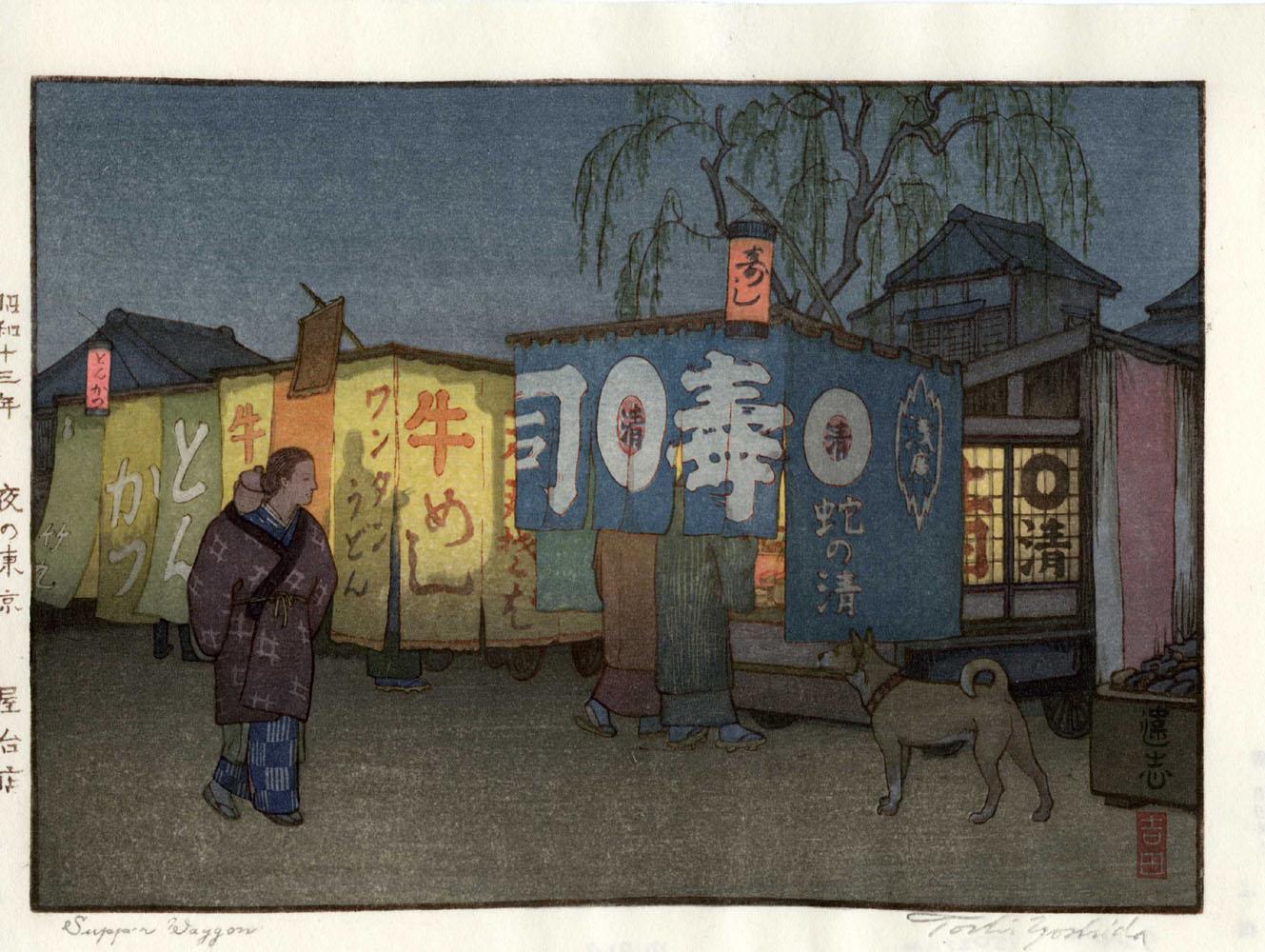This captivating image features a traditional Japanese painting, possibly a watercolour, with intricate ink detailing. The scene depicts a bustling nighttime marketplace, illuminated by lanterns and the warm glow from building windows. Japanese figures, adorned in kimonos, can be seen exploring various market stalls with rice paper coverings and screens bearing Japanese symbols and calligraphy. A brown dog with an orange collar sits attentively in the lower right corner, observing the activity. The sky, transitioning from blue to a deep night hue, frames the thin black-bordered artwork. On the far left, vertical Japanese text likely serves as the title, adding to the authenticity of this culturally rich piece.